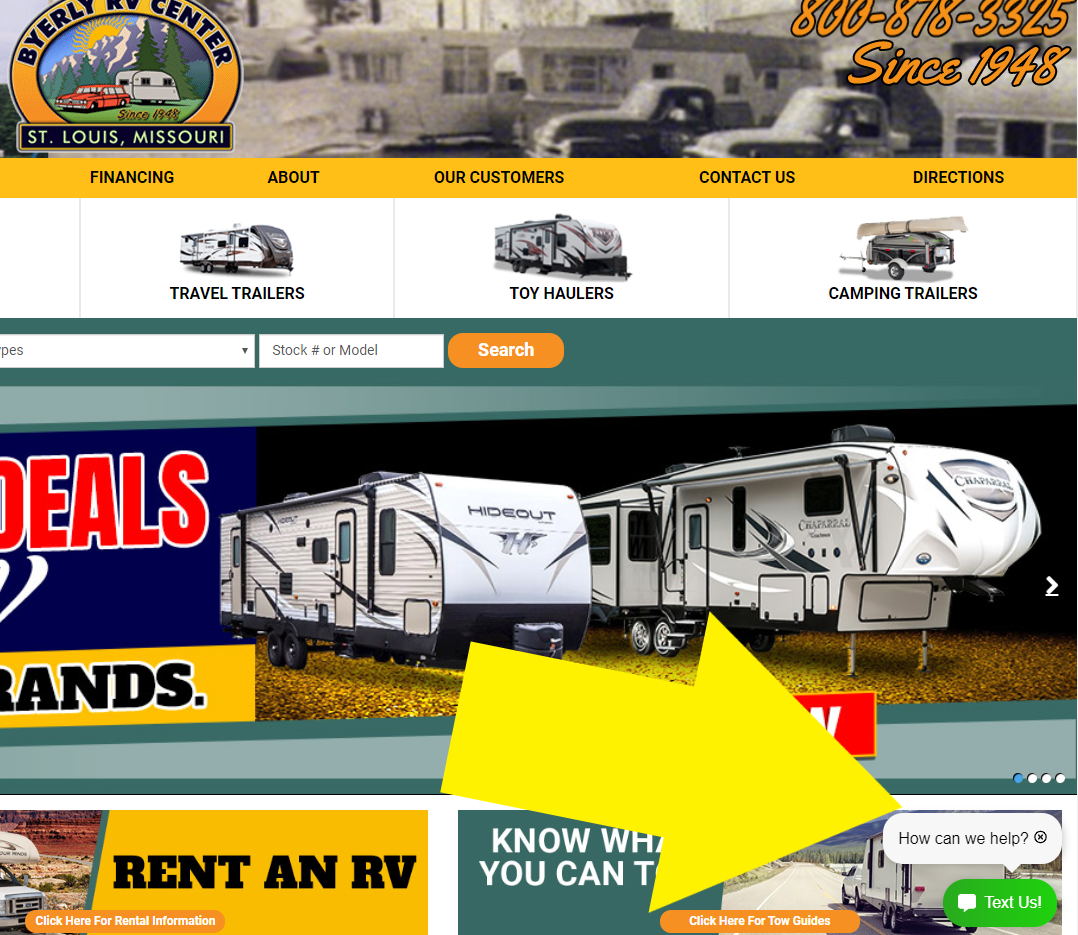The webpage for Beverly RV Center, located in St. Louis, Missouri, features a nostalgic black-and-white background at the top showcasing vintage trucks and trailers. In the top left corner, the company's name, "Beverly RV Center," along with the location, St. Louis, Missouri, is prominently displayed. This section also includes the business's phone number and a note indicating it has been operating since 1948.

Immediately below this, a bright yellow horizontal menu offers navigational options in bold black text, including "Financing," "About," "Our Customers," "Contact Us," and "Directions." 

Further down, on a white background, users can explore different categories such as "Travel Trailers," "Toy Haulers," and "Camping Trailers." Below these categories is an image displaying two campers, accompanied by a search bar for locating specific stock numbers or models.

In the bottom left corner, "Rattan RV" is written in black text on a yellow background. In the opposite corner, a white chat bubble labeled "How Can We Help?" invites user interaction, which is emphasized by a large yellow arrow pointing directly at it from the left.